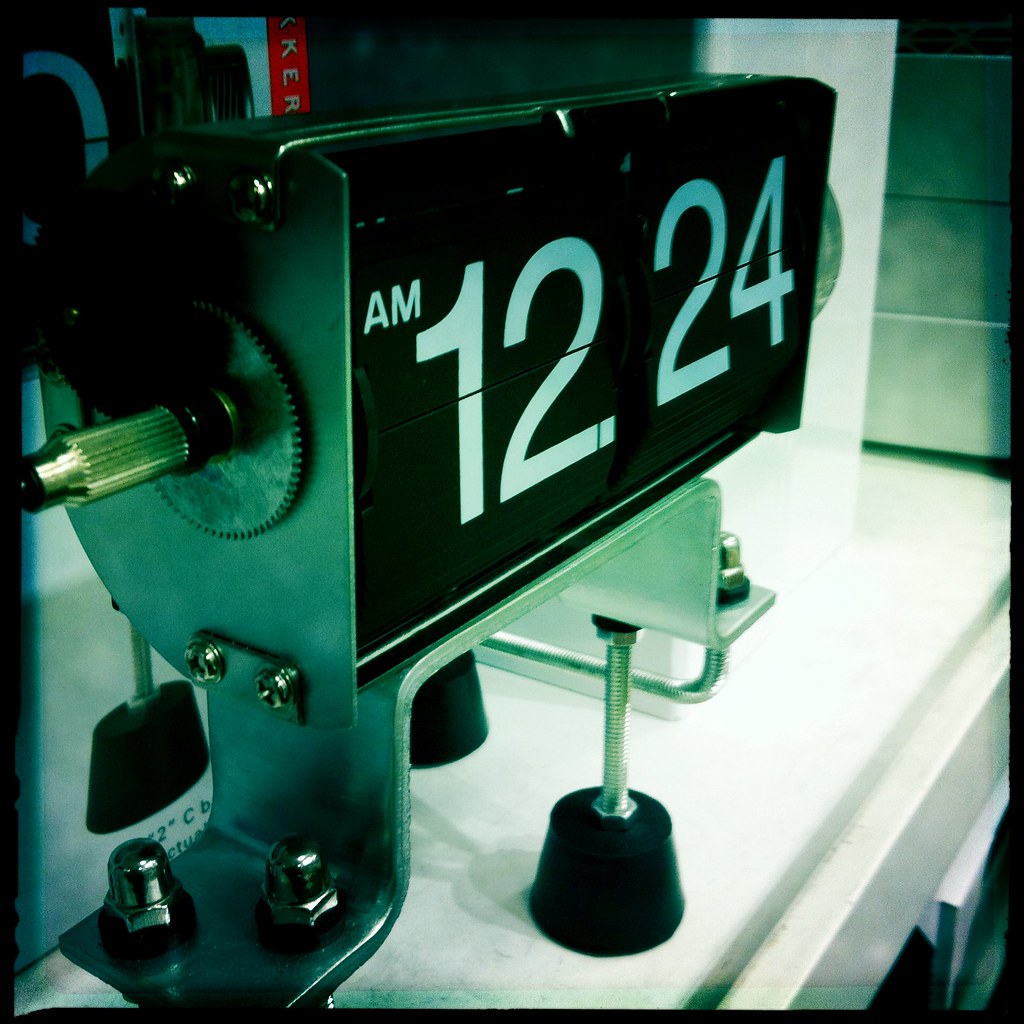This photograph features an industrial-looking clock prominently displayed in the forefront, mounted as if it's a tool with rubber feet. The clock is bolted onto a long, white metallic structure, and it has a black face with white text that reads "a.m. 12 24." The clock displays the numbers on separate squares, suggesting a mechanism where the hour and minute squares roll to change the time.

The background is somewhat cluttered, featuring metal paneling to the right and a white rectangle in front of it. To the upper left, there is a poster with a graphic that has a red edge. The surroundings appear to be in a room with walls made of rectangular cement bricks, enhancing the industrial ambiance of the scene.